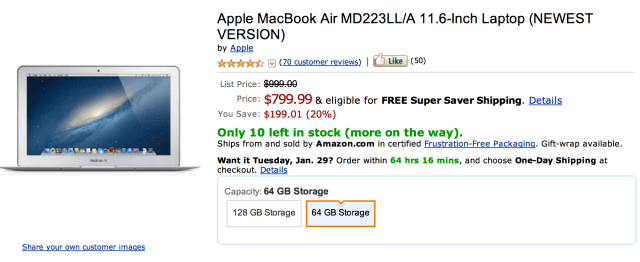Here is a cleaned-up and detailed descriptive caption for the image described:

---

The image is a screen capture featuring a product listing for an Apple MacBook Air MD223LL-A 11.6-inch laptop, the “newest version.” To the left of the screen, there is a visual of a white MacBook, which appears dated with its thick bezels. The MacBook is displaying a serene blue nature-themed wallpaper, and several icons are visible at the bottom of its screen. Below the MacBook image, there is a blue text prompt encouraging users to "share your own customer images."

Moving to the right of the screen, various textual details about the MacBook are presented in a mix of font colors. The product name and specifications are listed in black, blue, red, and green fonts. It indicates that the laptop is by Apple and has received an impressive rating of four and a half stars from 70 customer reviews, accompanied by 50 likes. 

The listing price, originally higher, is shown on sale for $799.99, with a note in red affirming a $199.01 discount or 20% savings. Blue clickable text offers more details about the pricing. The listing indicates that the product is eligible for free super saver shipping.

Beneath this, a green notification announces only "10 left in stock," with more units "on the way." The page confirms that the product ships from and is sold by Amazon.com, with a "certified frustration-free packaging" label. There is an option for gift wrapping, and an urgency note indicates that one-day shipping is available if orders are placed within 64 hours and 16 minutes, targeting a delivery by Tuesday, January 29th.

At the bottom, there is a blue button for further details near a section highlighting storage capacity options. The selected storage option is 64 gigabytes, colored in blue and orange, with an alternative 120-gigabyte option available but not selected.

---

This detailed caption provides a comprehensive overview of the visual and textual content presented in the screen capture.